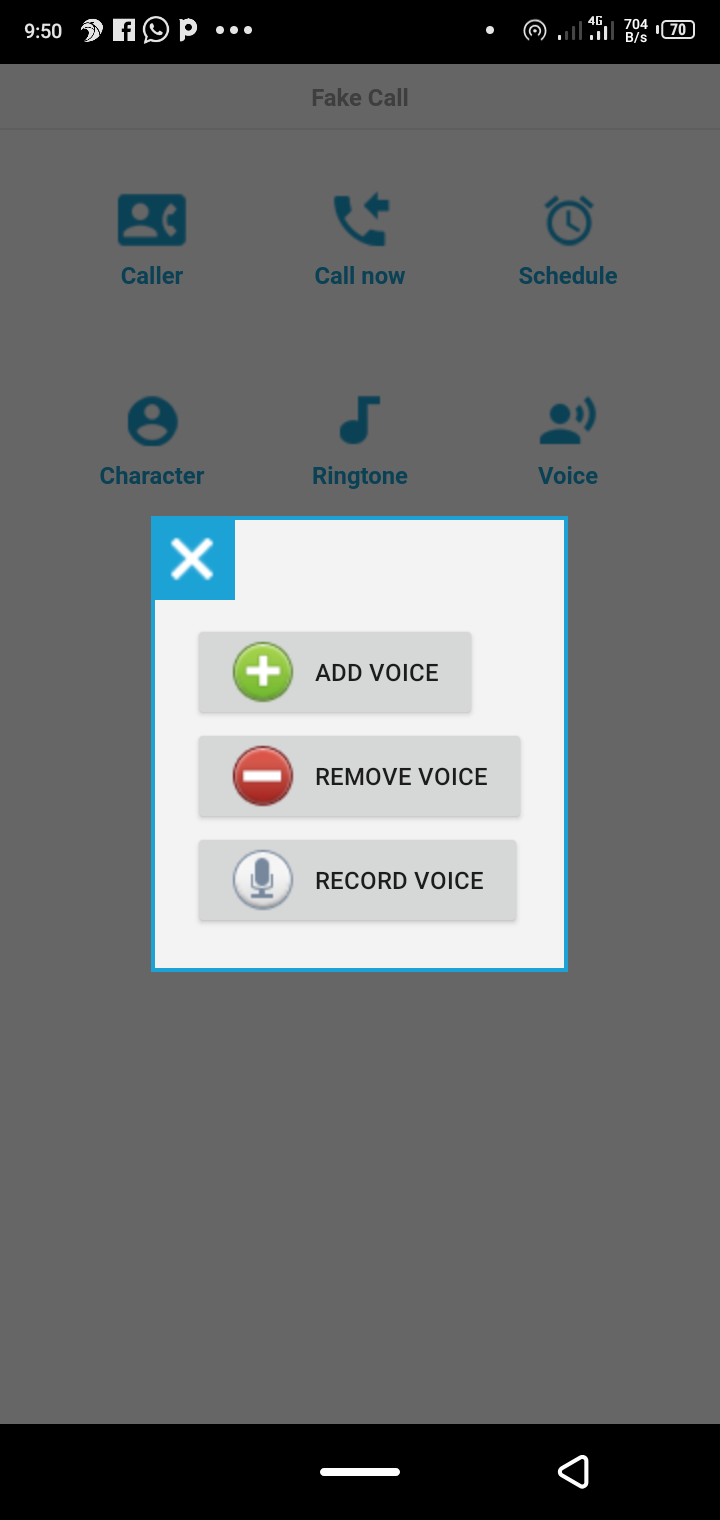A detailed smartphone screenshot showcasing a 'Fake Call' app interface. The screenshot has a faint gray overlay. At the very top, a black border displays a 9:50 timestamp, with a series of icons to the right: Facebook, WhatsApp, Pinterest (or a similar app), followed by three horizontal white dots, another unidentified white dot, an icon featuring three concentrically curved lines, a 4G Wi-Fi icon, and a battery icon showing 70% charge. Below the timestamp, the indicators show "704" with "B/S" beneath it.

The main screen under the gray overlay displays 'Fake Call' and several feature icons: 'Caller,' 'Call Now,' 'Schedule,' 'Character,' 'Ringtone,' and 'Voice.' 

A pop-up box on the screen labeled 'Add Voice,' features a green circle with a white plus sign and 'Remove Voice' with a red circle and a subtraction symbol. Below these is a microphone icon within a circle next to the text 'Record Voice.'

At the bottom, the black border houses two navigation buttons: a home button on the left and a left-facing arrow on the right.